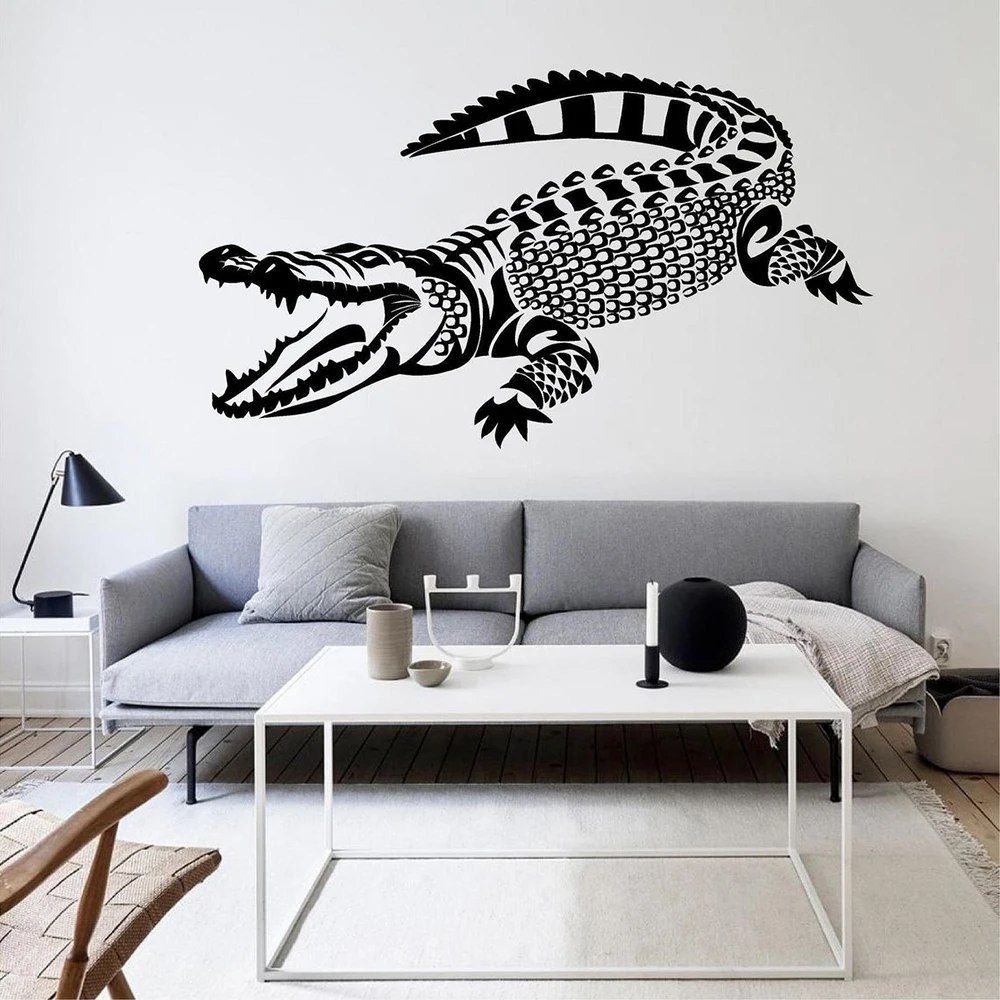The image showcases a modern living room with a minimalist design, dominated by a central gray couch adorned with a pillow on the left and a blanket on the right. Directly in front of the couch sits a stark white, square coffee table featuring a small collection of items, including a gray mug, a small gray dish, a black vase, a gray vase, a small gray bowl, a white candle with a black holder, and a large black ball. The floor beneath the coffee table is accented by a gray rug. In the foreground, the right corner of a brown, wooden chair is visible. Adjacent to the left of the couch, a small white end table supports a black lamp. The backdrop of the scene is a dual-toned gray wall, lighter on the left and darker on the right. Dominating this wall, directly above the couch, is a highly detailed, black-outlined stenciled depiction of a crocodile, stretching accurately from its open mouth on the left to its tail on the right, reminiscent of a graphic design or vinyl wall art. The arrangement and details suggest a carefully curated space, possibly featured in a design catalog or a website specializing in home decor or graphic artwork.